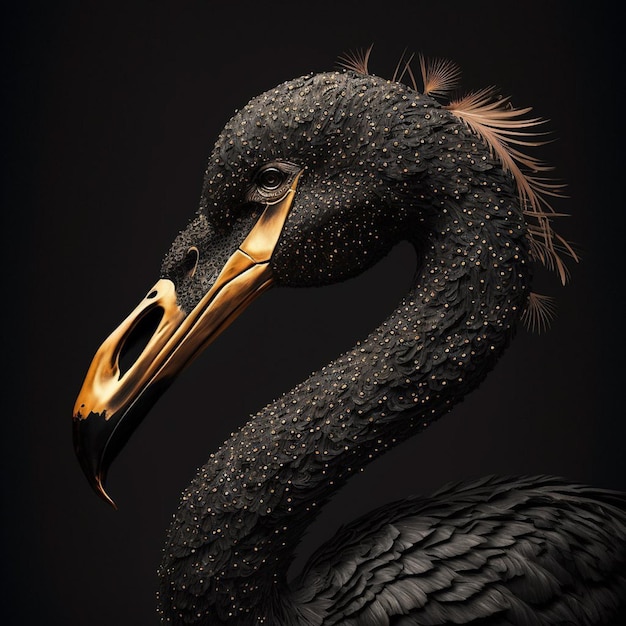This close-up image captures a fascinating bird that bears a resemblance to a swan, possibly a black swan. The focus is on the bird's long neck, which is predominantly black but adorned with small white spots or bumps. The intricate texture of these spots remains unclear even upon zooming in. The bird's head, viewed in a side profile facing left, features two blackish-brown feathers protruding from the top. Its eyes are a deep black, and the beak starts with a touch of black near the face, transitioning into a striking gold color, and ending with a black tip. The upper part of the bird's body, though partially visible, displays black feathers. Complementing the bird's dark plumage is a black background, which enhances the detailed and striking elements of its appearance.